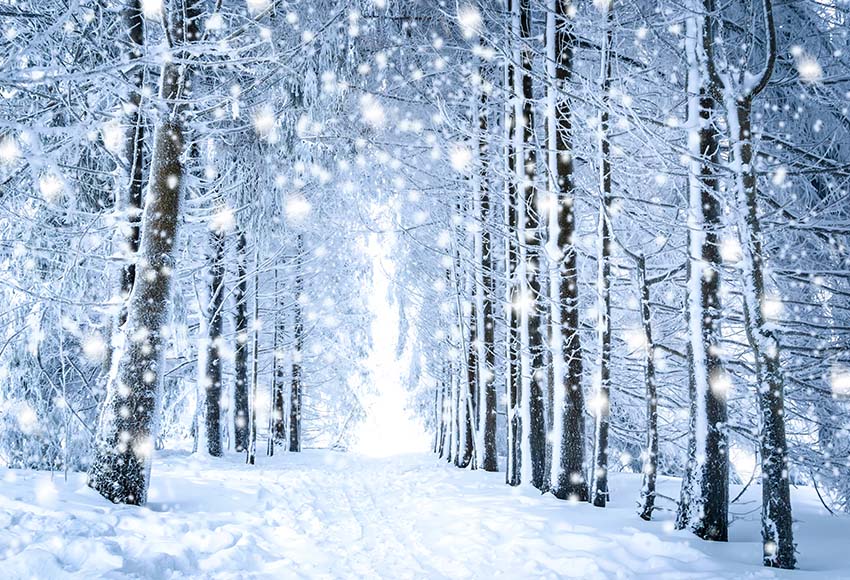This detailed digital illustration portrays a serene, snow-covered road flanked by tall trees on both sides, creating a natural corridor. Heavy snowfall is depicted throughout the scene, with large chunks of snowflakes cascading down. The trees, laden with snow, form a stark contrast against the bright, illuminated backdrop that extends into the horizon, giving a sense of depth and light. The path, devoid of trees, appears to ascend slightly towards the end of the image, reinforcing the perspective. Rendered primarily in shades of blue and white, the image captures the chill and tranquility of a snowy day, with the black tree trunks providing striking vertical accents. The overall composition is notably wider than it is tall, emphasizing the expansive wintry landscape.